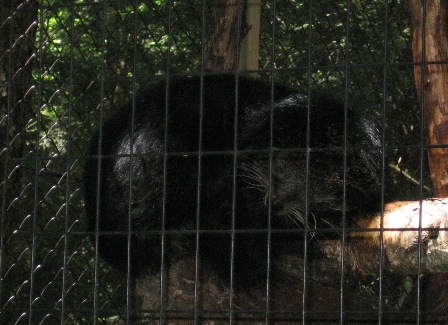In this detailed image of a zoo enclosure, a large, mostly white animal is barely discernible as it rests peacefully. Appearing to show its backside, the animal is perched on a brightly sunlit wooden log, its head tucked into its chest, eyes seemingly closed, suggesting it is asleep. The fencing in the foreground comprises two different types: the left third is a diamond-shaped crisscrossing of metal chain link wire, while the other two-thirds consists of sturdier metal bars arranged both vertically and horizontally. The enclosure is shrouded in shade, with the background displaying an assortment of lush tree leaves and branches. There are also two prominent tree trunks: a greenish one centrally located and a more traditional wooden brown one to the right. The setting hints at additional climbing structures, reinforcing the likelihood that this is a zoo habitat designed for the animal's enrichment and comfort.